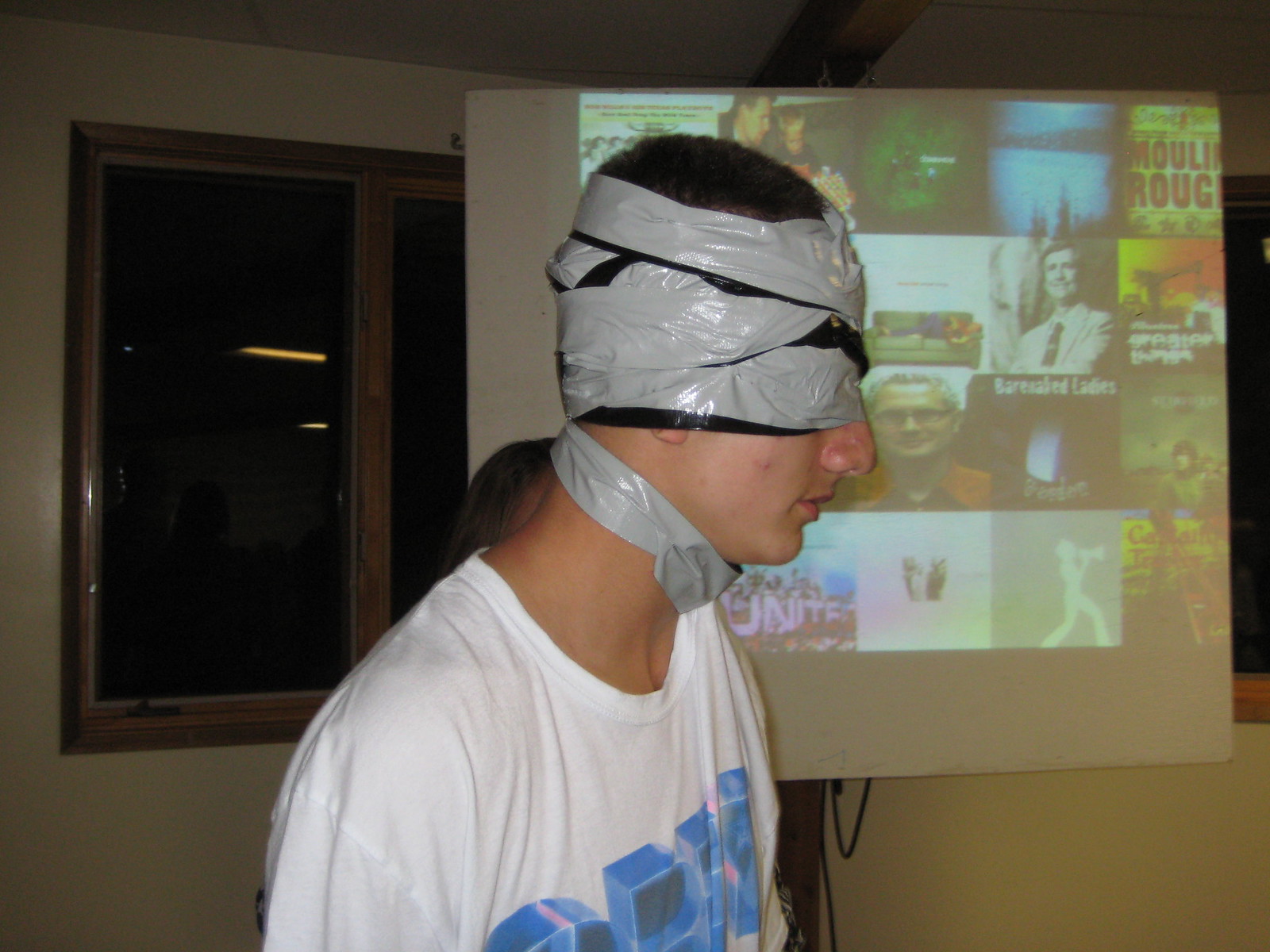The image depicts a young Caucasian man, likely in his late teens to early twenties, with long hair pulled back in a ponytail. He is wearing a white t-shirt with blue lettering and is shown in right profile, situated towards the center of the photo. His face, head, and neck are extensively wrapped in shiny black and gray tape, resembling duct tape and possibly electrical tape, with a strip of black plastic bag or similar material underneath to prevent direct contact with his skin. The tape covers his eyes and forehead completely, extending partially over his nose and most of his ears, leaving his nostrils, mouth, and chin exposed. Around his neck, there is an additional piece of tape that looks like a collar. 

In the background, on the left side of the photo, there is a dark sliding window with brown wooden frames, reflecting light and faint images of people. Behind him is a white screen that appears to be projecting rows of square images, which are likely album covers or movie soundtracks. Among these, visible titles include "Moulin Rouge," with the text "Songs From" or "Soundtrack," and "Bare Naked Ladies."